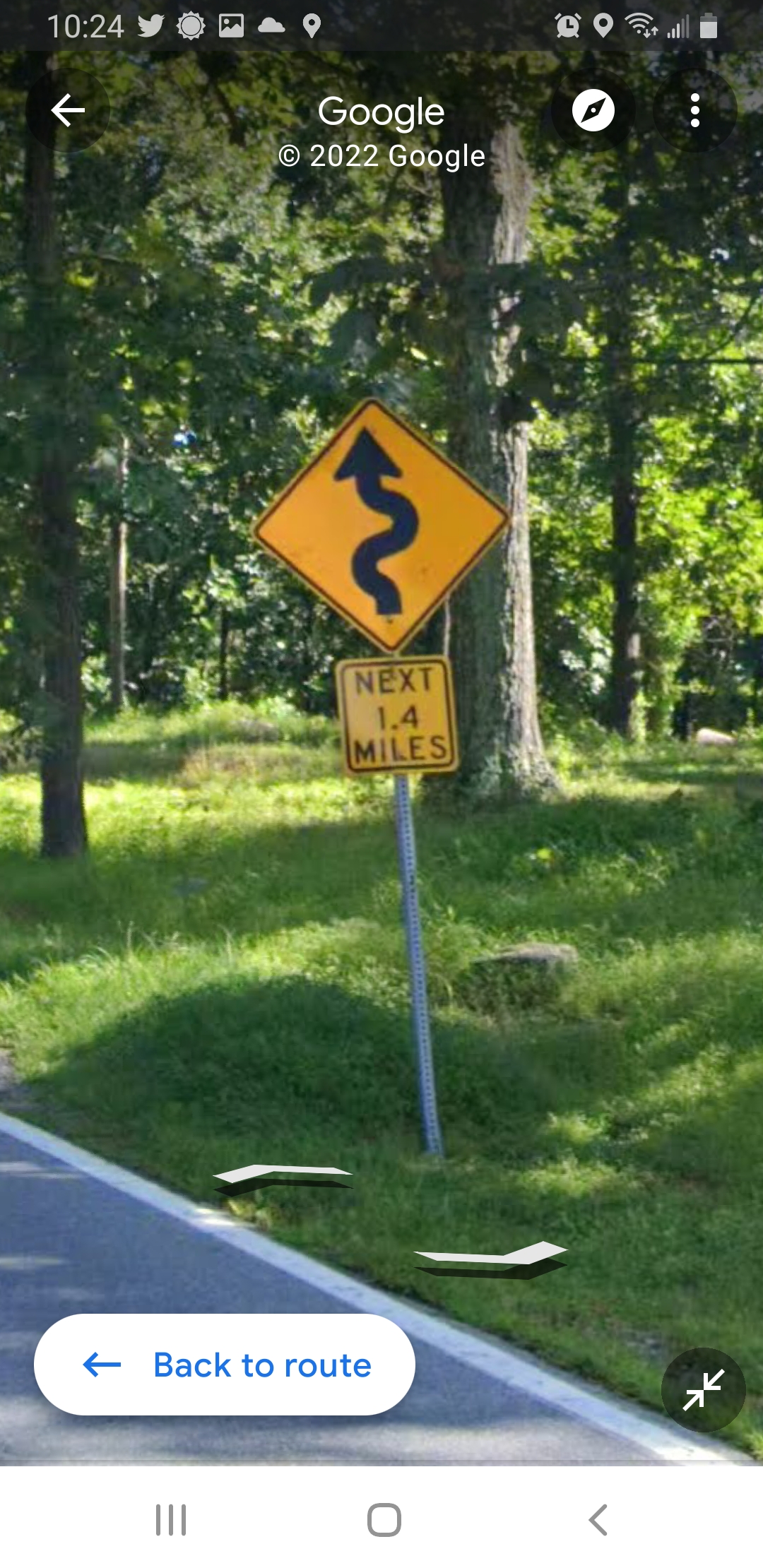The image is a screenshot from Google Maps Street View captured on an Android phone at 10:24 a.m., as indicated by the icons for Twitter, alarm, battery, and signal strength at the top. The Google and copyright 2022 Google label is also present at the top. The focus of the screenshot is a roadside sign positioned on a silver pole in a partially wooded area with two big trees and some grass. The sign consists of two yellow signage elements: a larger diamond-shaped sign at the top featuring a black curved road symbol, indicating winding roads ahead, and a smaller square sign below it stating "Next 1.4 miles" in black text. At the bottom left corner of the image, there is a "Back to route" button with an arrow pointing left. The image appears slightly blurry and shows the greenery of the trees dominating the background, with only a small portion of the road and its side markings visible.